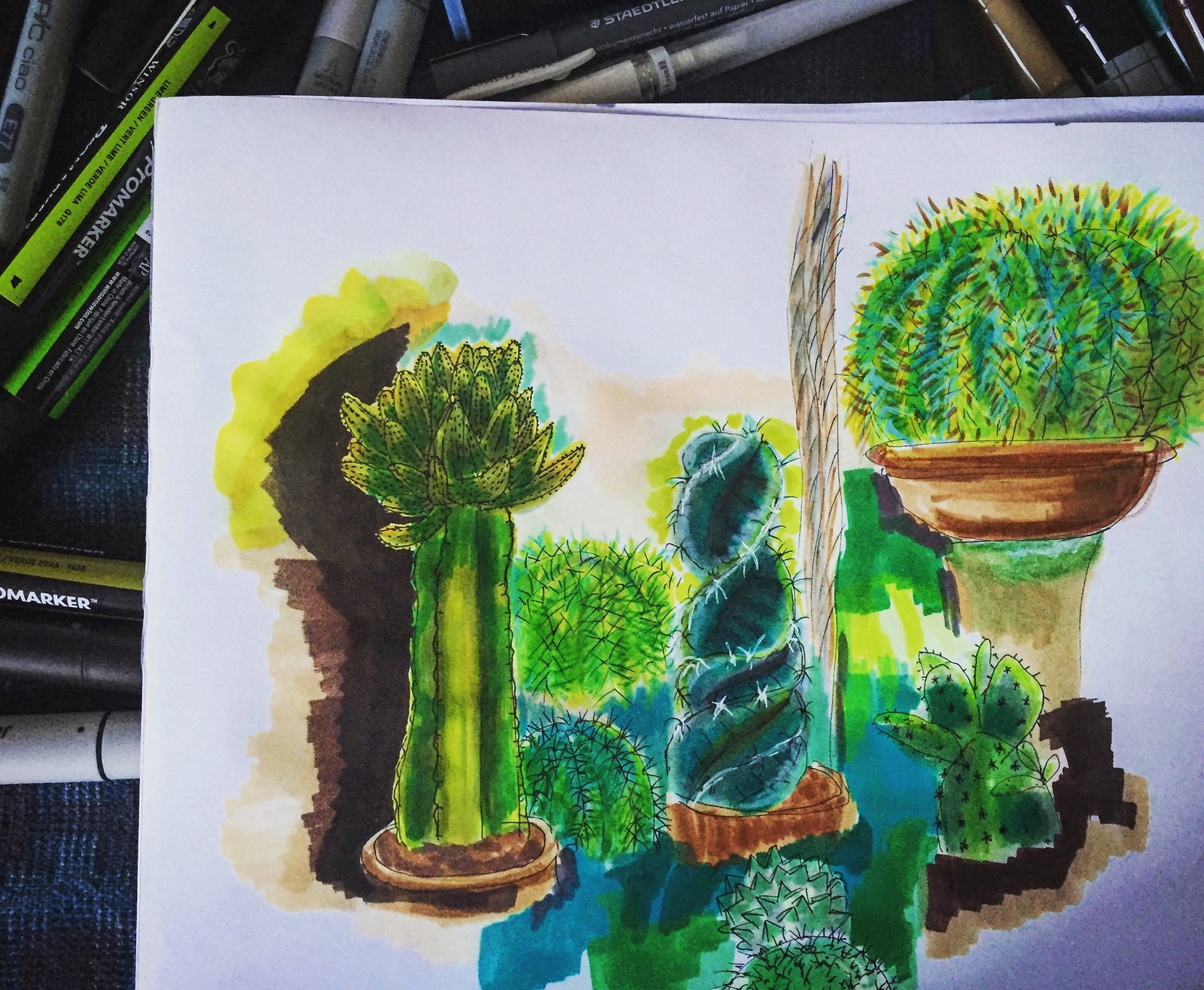This image showcases an artwork displayed on white sketch paper, lying atop a blue surface filled with assorted pens, markers, and watercolor markers scattered in an L-shape from the top right to bottom left. The artwork, rendered in various shades of green and yellow-green markers and pens, depicts an array of succulent plants and cactuses. On the left, a prominent cactus with a large, spiky bloom is depicted without branches. Adjacent to it, two tiered bushes add layered complexity, and further right, a spiral-shaped green form wrapped in what appears to be barbed wire leads to a distinctive pineapple-shaped bush. Another cactus nestles towards the bottom left, and nearby, a spiky bush sits atop a pedestal capped with a brown bowl. The plants are delicately shaded with brown hues and accented with pen-drawn spikes, giving the foliage a vibrant, almost glowing appearance.